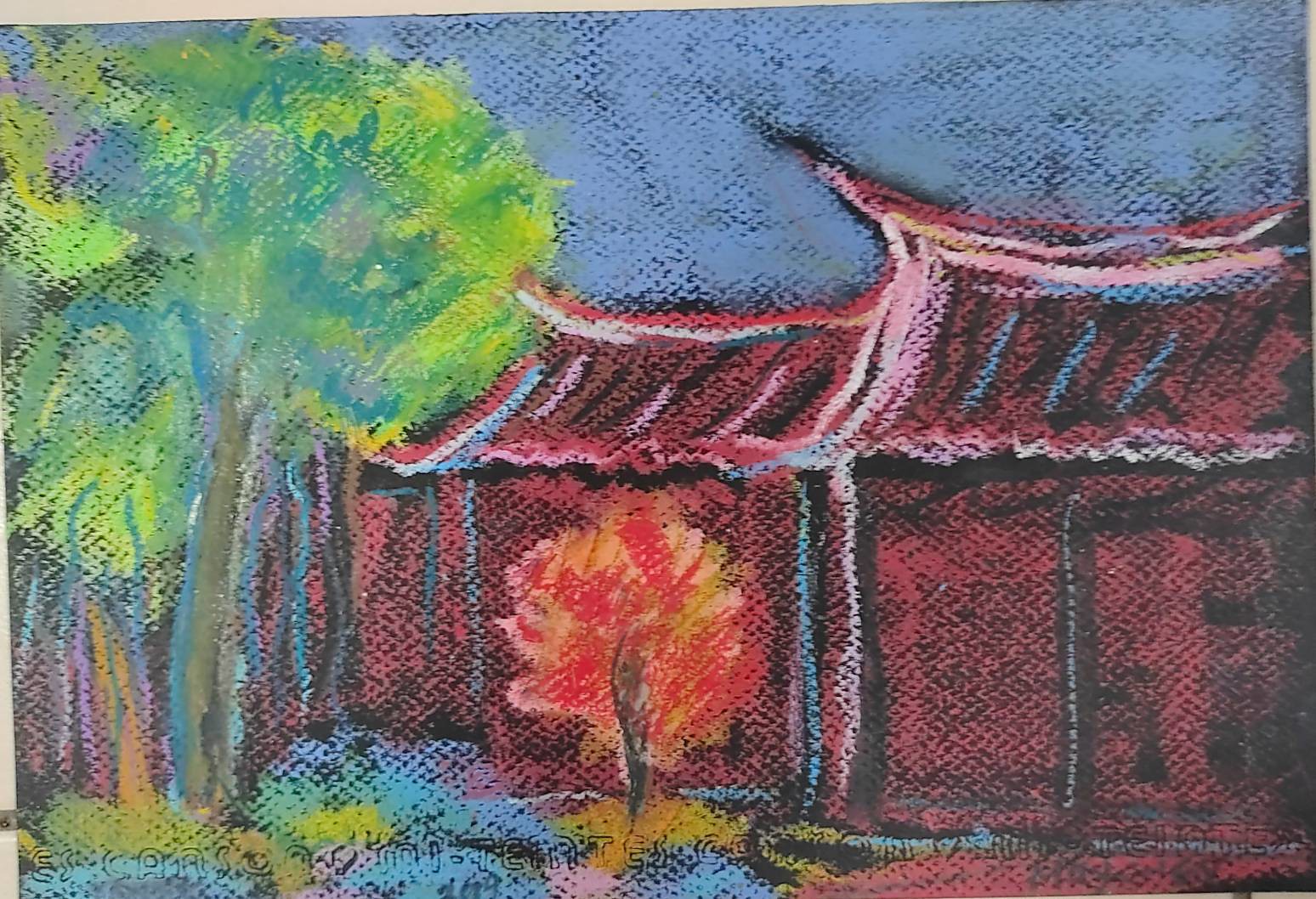The image appears to be a vibrant and textured pastel or watercolor drawing depicting an oriental-style, single-story cabin with ornate, pagoda-like roofs. The building, which is situated prominently from the center to the right edge of the image, features an intricate roof structure with pointed peaks extending outward. It is rendered in shades of brown with distinctive white highlights accentuating the edges of the roof and columns. Foreground elements include a striking reddish bush, painted in rich hues of red, orange, and brown, positioned in the lower center. To the left of the scene stands a tall tree, about a story and a half high, which is illustrated with a brown trunk and leaves shaded in varying tones of light and dark green interspersed with blue lines. The upper portion of the image, particularly to the right of center and extending to the right edge, showcases a clear blue sky. An indiscernible text overlay spans the bottom of the image from left to right, adding a mysterious element to the artwork.